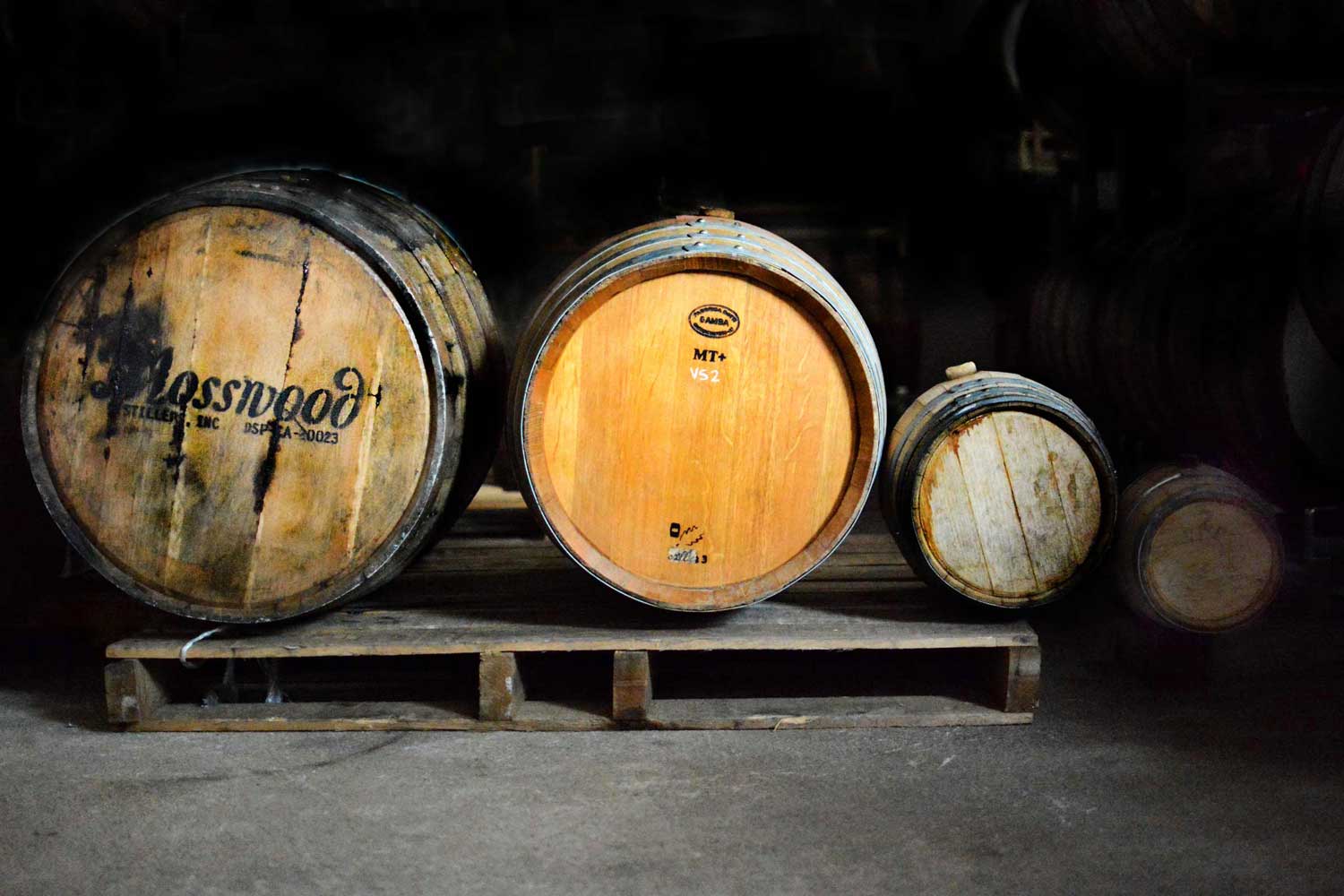The image depicts four wooden barrels, likely used for storing wine or whiskey, situated within a dimly-lit, possibly old warehouse. Three of the barrels rest on a weathered wooden pallet with chipped edges, while the fourth lies on the concrete floor, suggesting they might have once been tied together and have since come undone. The barrels vary in size and condition. The largest one on the left features the text "moss wood" in an italic black font. The barrel second from the left appears to be the freshest and brightest, in contrast to the others that show signs of wear and age. One of the barrels bears a bright color with dark black text reading "MT" on its yellow section. The overall lighting highlights the foreground of the barrels, possibly from natural light filtering through a window or artificial studio lighting, enhancing the details and textures of the scene.